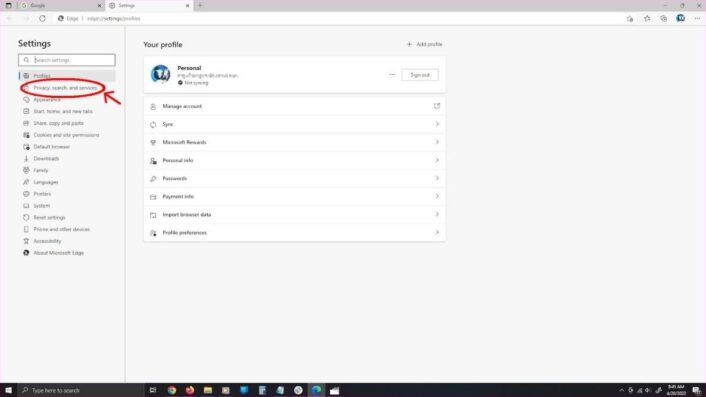A low-resolution screenshot of a computer screen displaying the settings page of the Microsoft Edge browser on a Windows operating system. The image is focused on the "Privacy, Search, and Services" section, which is accentuated with a red circle and a red arrow for emphasis. To the right of this highlighted area is the "Your Profile" section, featuring options such as "Add Photo," "Personal Account," "Manage Account," "Sync," and "Microsoft Rewards," although the text is blurry and difficult to read. The Windows taskbar is visible at the bottom, featuring icons for Google Chrome, Firefox, and File Explorer among others. The screenshot is captured in a widescreen landscape format.